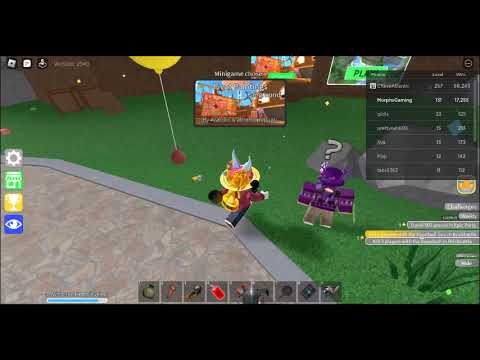This image captures a detailed scene from a Roblox mini-game. Two characters with the distinctive boxy bodies characteristic of Roblox are running through a world with both grassy and concrete terrains. The character on the left is outfitted in a red outfit, sporting a yellow hat with blue horns and a lava-like decoration on the forehead, appearing to run toward the bottom left. To the right is a more robot-like character with a squarish, purple top half, a robot helmet and shoulders, white text on their chest, and white pants. This character is emitting a question mark symbol. The upper left-hand corner of the screen features a silver Roblox icon, confirming the game's identity.

In the bottom corner, a blue bar likely indicating stamina or health is visible, contrasting against nine gray squares with items, suggesting an item menu. A brown house with some sort of mural or design on it is noticeable behind the characters along with a tall balloon secured by a brown sack. Meanwhile, on the bottom, a scoreboard in black with usernames in white text is positioned in the upper right-hand corner, tracking the players' scores.

An assortment of symbols including settings, home, trophy, and eye icons are visible on the left side of the screen, indicating various game options. The surrounding environment also shows elements like tall weeds and perhaps a sandbox, while the white wall with pictures adds depth to the setting, creating an engaging and vividly depicted virtual scene.